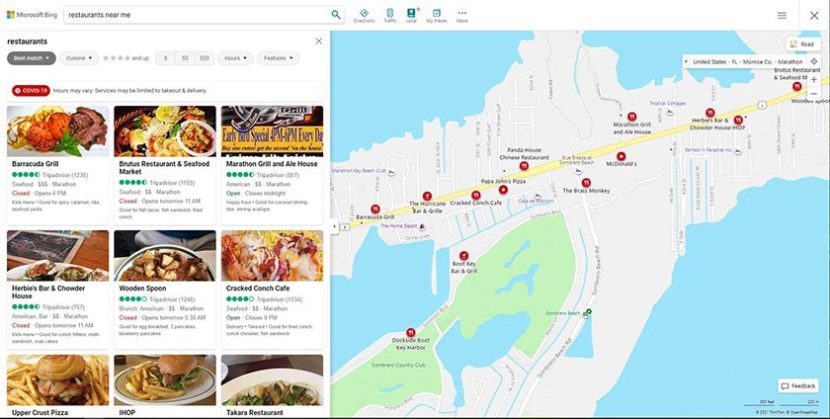A small, low-quality desktop image shows a user interface likely running on a Windows operating system, identifiable by the Microsoft Bing logo prominently displayed on the web browser or search engine. The user seems to be searching for "restaurants near me." Alongside the search bar, various icons are visible, indicating options such as directions (depicted by a road sign), traffic updates (shown with a traffic light), a small book icon with a red asterisk (text unreadable), a checkmark labeled "My Favorites," and an ellipsis for more options. Further to the right, there's a hamburger menu for additional settings and an exit option.

The results page displays the search term "restaurants," with filter and sorting options in gray text, suggesting categories like "Best Results" and "Cuisine." Users can filter results by star ratings and adjust the number of visible entries from two to six at a time. The page includes details like restaurant hours, which might be affected by COVID-19 restrictions, indicating varied hours and limited services to takeout and delivery.

Listed are multiple restaurants, each with names, types of cuisine, price estimates, and TripAdvisor ratings. Displayed restaurants include Barracuda Grill, Brutus Restaurant and Seafood Market, Marathon Grill and Ale House, Herbie's Bar and Chowder House, Wooden Spoon, Cracked Conch Cafe, Upper Crust Pizza, IHOP, and Takara Restaurant. The interface also features a map highlighting the locations of these dining options. Overall, it's clear that someone is using Microsoft Bing to search for nearby restaurants.